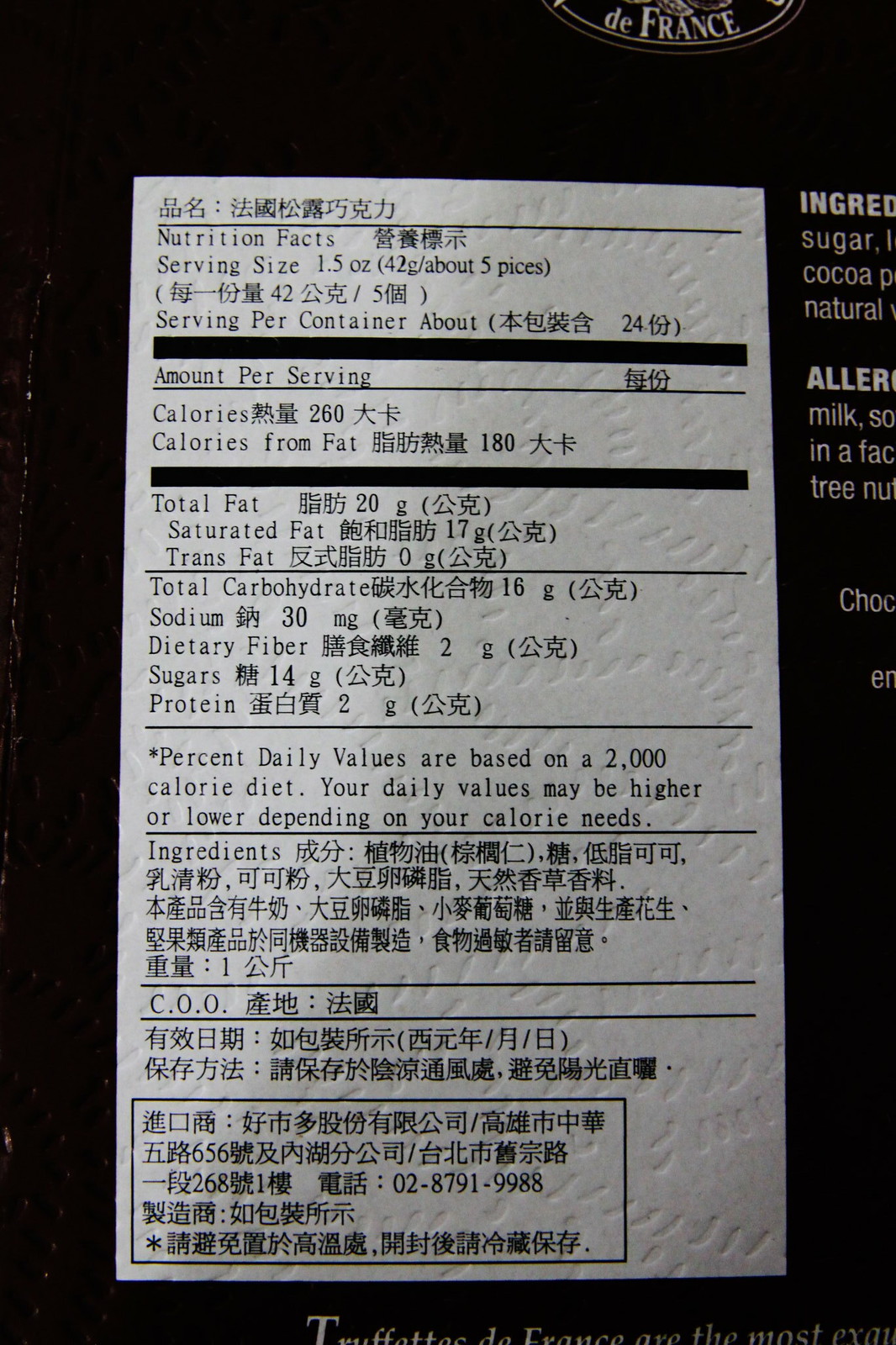This detailed caption provides an in-depth description of a nutritional information label found on the back of a box. The label is presented on a vertically-oriented white rectangle, featuring nutrition facts listed in both English and Japanese. These include serving size, servings per container, amount per serving, calories, calories from fat, total fat, saturated fat, trans fat, total carbohydrate, sodium, dietary fiber, sugars, protein, and a note that percent daily values are based on a 2,000 calorie diet. It mentions that daily values may vary based on individual calorie needs.

Below the nutritional data, the label lists the ingredients entirely in Japanese, unlike the nutritional content which is bilingual. Interestingly, the section entailing ingredients and everything else below it is not translated into English. It features a portion labeled "COO" followed by Japanese characters, after which all subsequent text remains in Japanese, indicating it is a foreign product or one aimed at a bilingual market.

Surrounding the white rectangle is a black box, suggesting the label is part of a larger packaging, presumably the box of the product. Towards the top right corner of the label, part of the ingredients section appears in English, with readable words like "sugar," "cocoa," and "natural," though they are partially cut off. Below this, beginning of an allergy information section is visible, with words like "milk," "soy," "factory," and "tree nut" discernible, pointing out possible allergen warnings.